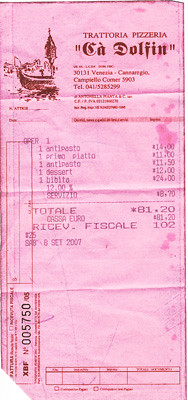Caption: 

This image features a pink receipt from Chatteria Pizzeria C.A. DOLFIN, written in a distinctive, medieval-style script. The receipt appears to be from a European restaurant, possibly located in Italy. The address is partly legible, showing "30134 Venezia," suggesting a location in Venice. There is an intricate graphic on the left side, which might represent something iconic to the city or the establishment.

The items ordered include antipasto, primaplata, antipasto (listed twice), dessert, and bibito, with a serving tip of 8.70 in an unspecified currency. The total amount on the receipt is 81.20, hinting that it is likely not in U.S. dollars. Additionally, there is a coded term, "RICEV. FICALE," valued at 1.02, and a ticket number "005750" is visible.

Despite the challenge in reading some parts of the receipt, it conveys a charming glimpse into a delightful dining experience at this European pizzeria.